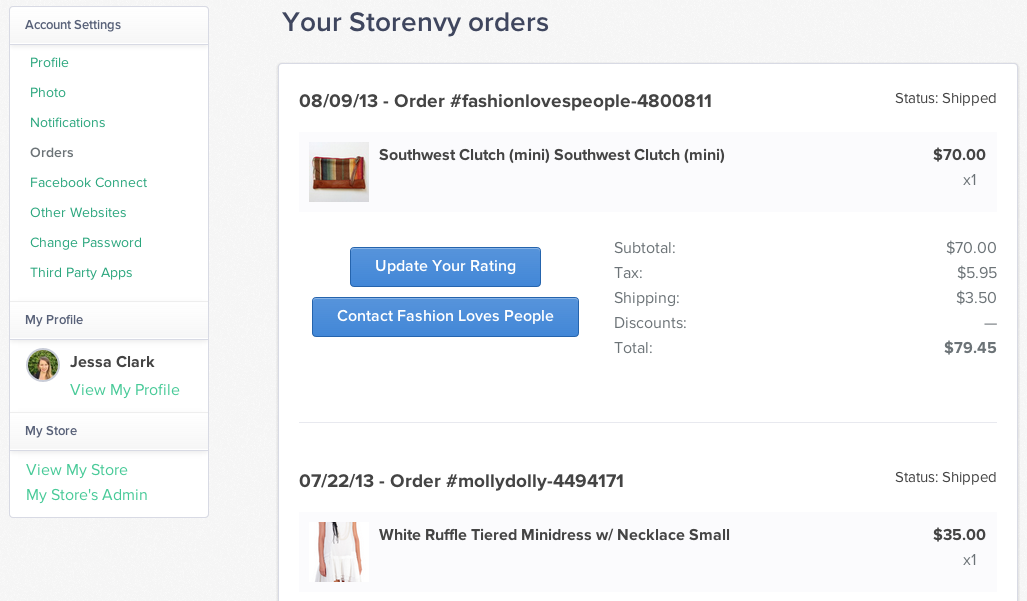### Detailed Caption for Image

The image is a screenshot of an order summary from the women's shopping site "Stormby." The account belongs to Jessa Clark, whose profile picture and name are visible on the left-hand side of the page. The top of the page features her profile photo, alongside options such as notifications, and a section titled "Your Stormby Orders," highlighting the current page. Only the "Orders" section is not highlighted in green, indicating it is the active section. Additional account options include Facebook connect, links to other websites, password settings, and permissions for third-party apps.

The order in question dates back to August 9, 2013, marked by the creative order hashtag "fashion loves people" along with a specific order number. The order status is "Shipped."

1. **Item 1**: Southwest Clutch Mini
   - **Description**: A compact clutch purse, although the image doesn't clearly resemble a purse.
   - **Price**: $70
   - **Quantity**: 1
   - **Subtotal**: $70
   - **Additional Costs**:
     - **Tax**: $5.95
     - **Shipping**: $3.50
   - **Total Cost**: $79.45

2. **Item 2**: White Ruffle Tiered Mini Dress with Necklace
   - **Description**: A small-sized mini dress, resembling a tennis dress with white ruffles.
   - **Price**: $35

Both items have successfully shipped. The total order cost sums up to the detailed amounts provided.